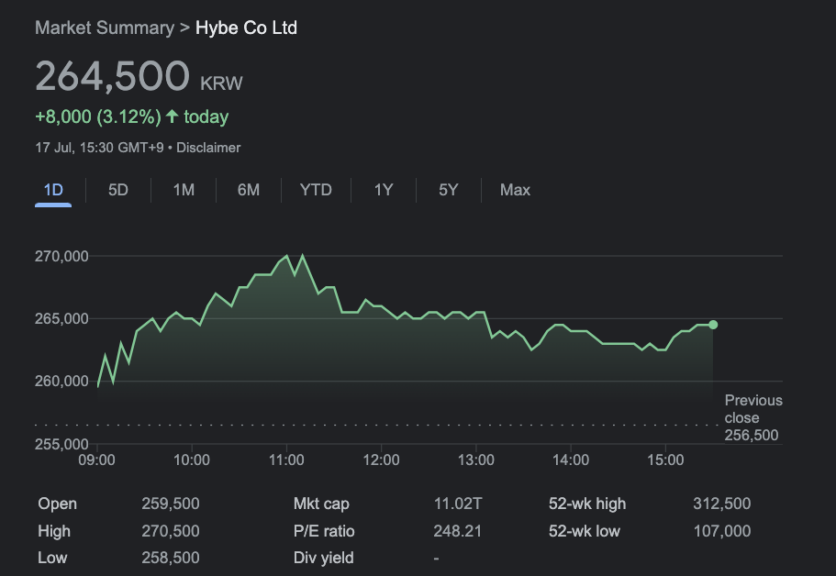A detailed screen capture from a financial website provides a daily market summary for Hybe Co Ltd. Highlighting the current stock price at 264,500 KRW, the display indicates a positive change of +8,000 KRW, translating to a 3.12% increase for the day. The date and time, marked as July 17, 15:30 GMT+9, appear prominently alongside a standard disclaimer. The chart focuses on a one-day performance, showing that the stock price initially opened at 259,000 KRW and peaked at 265,000 KRW. A green line graphically illustrates the stock's upward movement throughout the trading day, reflecting various performance metrics and other pertinent data about the company's stock.